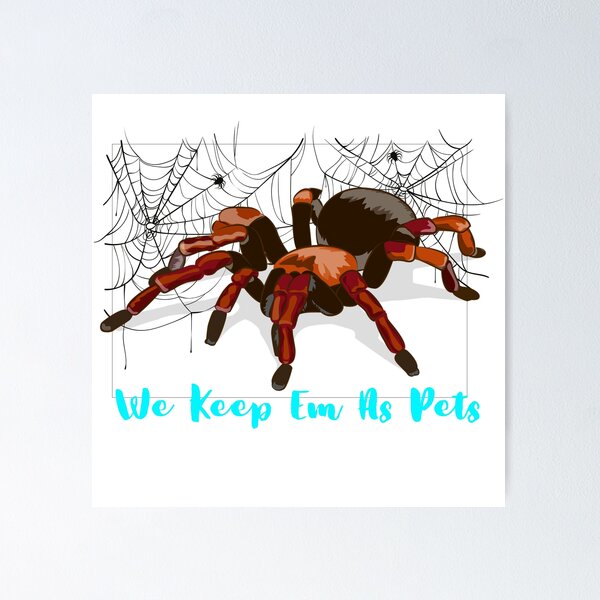The image is a detailed, stylized drawing centered within a grayish-white border. Inside a white square set against this border, a large, prominently featured tarantula is illustrated. The tarantula's body includes a variety of colors such as black, shades of brown, white, and gray, with its legs sporting red and black hues. Surrounding the central tarantula are two black spider webs, each hosting a tiny, cute black spider. Beneath the tarantula, blue text reads "WE KEEP EM AS PETS," suggesting an homage to spiders, possibly as an advertisement for keeping spiders, including tarantulas, as pets. The drawing is professionally executed with a well-detailed, cartoon-like quality, emphasizing the artistic and somewhat educational nature of the piece. The overall background surrounding the white square is gray, giving a clean and striking contrast to the detailed artwork within.